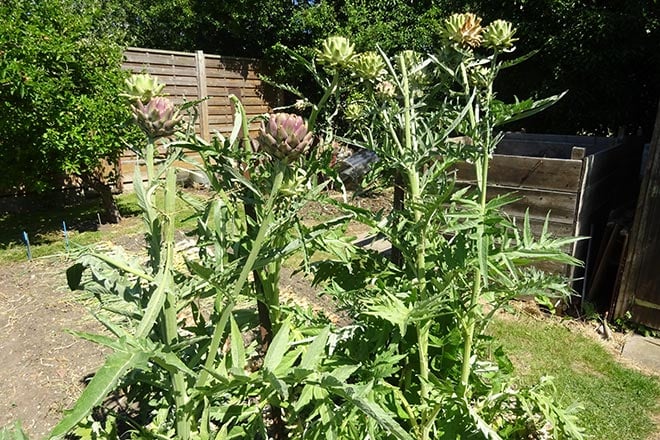This image captures an outdoor garden scene during the daytime. At the forefront, long, thick green stalks, approximately three inches wide and extending nearly to the top of the photograph, dominate the base. Adorning these stalks are serrated leaves that branch out to the left and right. Each stalk culminates in a budded or blooming flower, with petals characterized by a thick, almost succulent appearance. The petals vary in color, with some being a vibrant green while others exhibit a light purplish-pink hue.

The ground in this garden is mostly brown, suggesting dirt, though a sparse scattering of grass is visible on the right side. To the left, the ground appears ready for planting. In the background, the image includes verdant bushes located in the upper left corner, while a wooden fence spans horizontally across the scene, contributing to the rustic charm. On the far right, additional trees are visible along with what appears to be a wooden raised garden bed, further enhancing the garden's structured yet natural aesthetic.